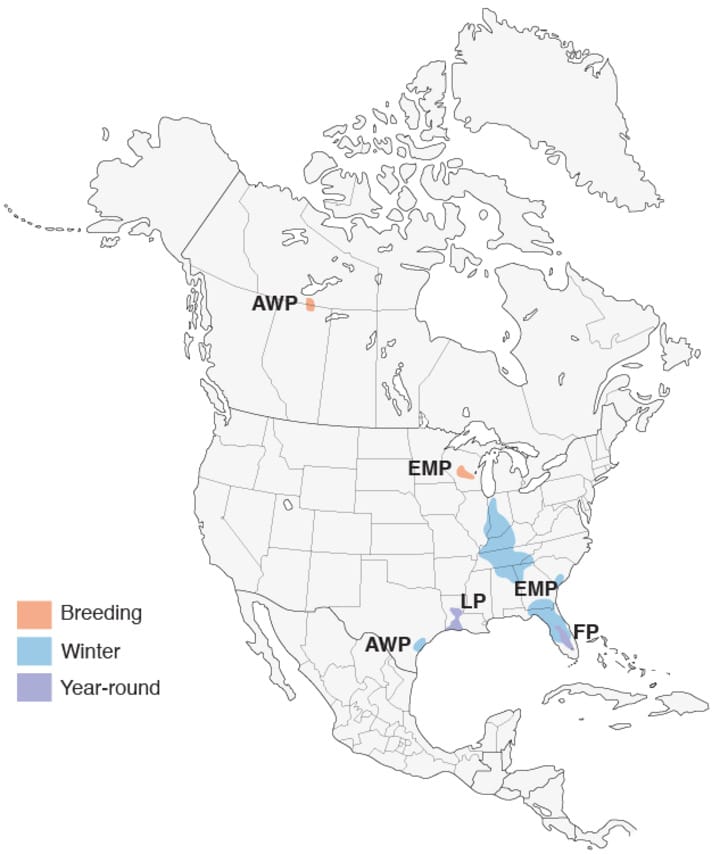This image depicts a detailed map of North America, covering Canada, the United States, and Mexico. The map features various dots and labels correlated by a key located on the left side, which includes three small squares in distinct colors: pink for breeding, light blue for winter, and purply blue for year-round.

In Canada, a pink dot labeled "AWP" signifies a breeding area. Within the United States, a pink dot marked "EMP" is seen in Minnesota, indicating another breeding site. Texas hosts a light blue dot named "AWP," representing a winter region. Louisiana displays a purply blue dot labeled "LP," indicating a year-round zone. Further, Georgia has letters "EMP," and Florida shows "FP."

The map encompasses not only the central landmass of North America shaded in light gray against a white background but also includes small islands and other detailed surroundings. The consistency in the dots and initials such as AWP, EMP, LP, and FP across the continent helps to illustrate specific geographical patterns and behaviors depicted by shades and labels.